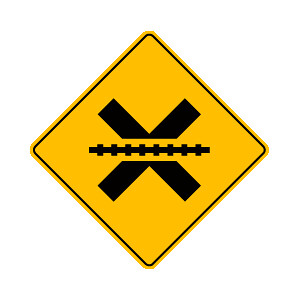The image depicts a diamond-shaped road sign with its points facing up, down, and to the sides, resembling a square rotated 45 degrees. The sign's background is caution yellow with a thin black border around the edge. At the center, a large black "X" is prominent, with a distinctive design featuring what appears to be railroad tracks running horizontally through its midsection. This horizontal element consists of a straight black line intersected by several short vertical lines, mimicking the appearance of train tracks. The sign's overall design is common for roadside indicators, serving as a warning for a railroad crossing ahead.